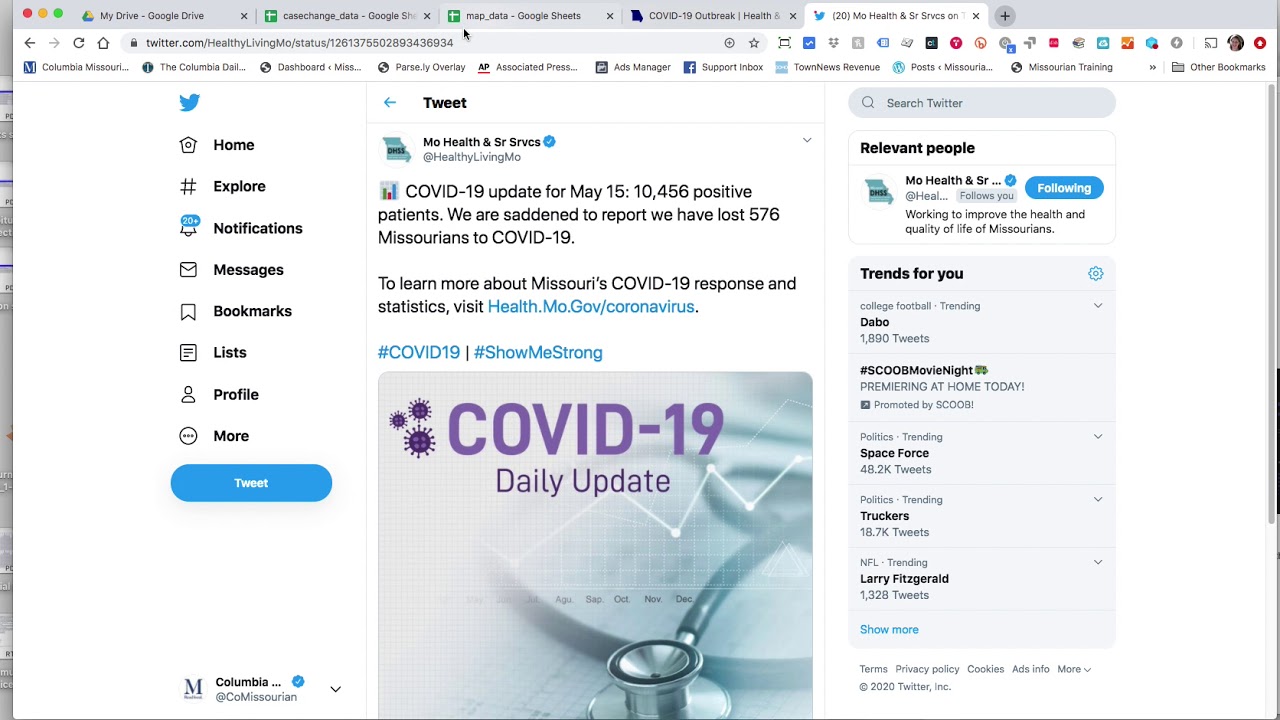The image is a screenshot from a website featuring various sections and a specific tweet related to COVID-19 updates. At the top of the image, the website menu shows options such as 'My Drive', 'Cash Exchange', 'Map Data', 'COVID-19 Outbreak', and 'MO Health and Senior Services.' 

In the central part of the image, there is an embedded Twitter feed with a tweet prominently displayed. The tweet, from 'MO Health and Services' under the handle 'Healthy Living MO', provides a COVID-19 update for May 15th. It reports that there are 10,456 positive cases in Missouri and that 576 Missourians have died from the virus. The tweet directs users to learn more about the state’s COVID-19 response and statistics at 'health.mo.gov/coronavirus.' 

Attached to the tweet is an image featuring a stethoscope and purple text that reads 'COVID-19 Daily Update.' 

On the right side of the screenshot, there's a section labeled 'Relevant people,' followed by a 'Trends for you' area with clickable topics, including categories such as truckers, NFL, and Larry Fitzgerald.